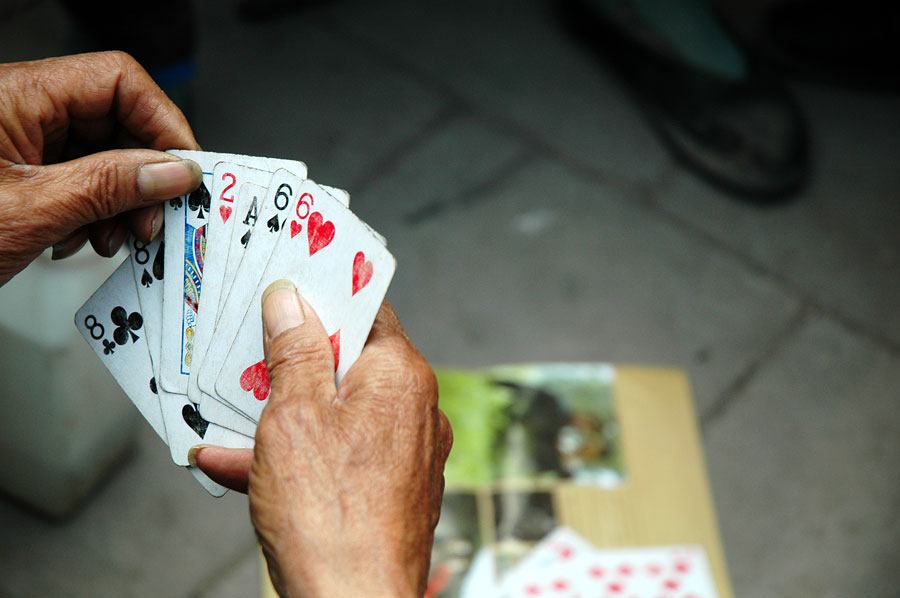In this evocative image, the viewer's attention is drawn to a pair of aged, wrinkled hands situated on the left-hand side of the frame, clutching a set of eight worn-out playing cards. The cards held by the elder include the eight of clubs, eight of spades, king of spades, two of hearts, ace of hearts, six of spades, and six of hearts. The lengthy and dirt-streaked fingernails add to the overall sense of weathered, enduring hands that have likely seen many games played out. The backdrop consists of a plain ground floor, with the presence of another pair of shoes indicating a second person partaking in the card game. Scattered around on the floor are additional stacks of cards and an open magazine, reinforcing the informal and impromptu nature of the setting. The image captures the essence of the moment—the simplicity of a timeless game shared in a humble, unadorned environment.